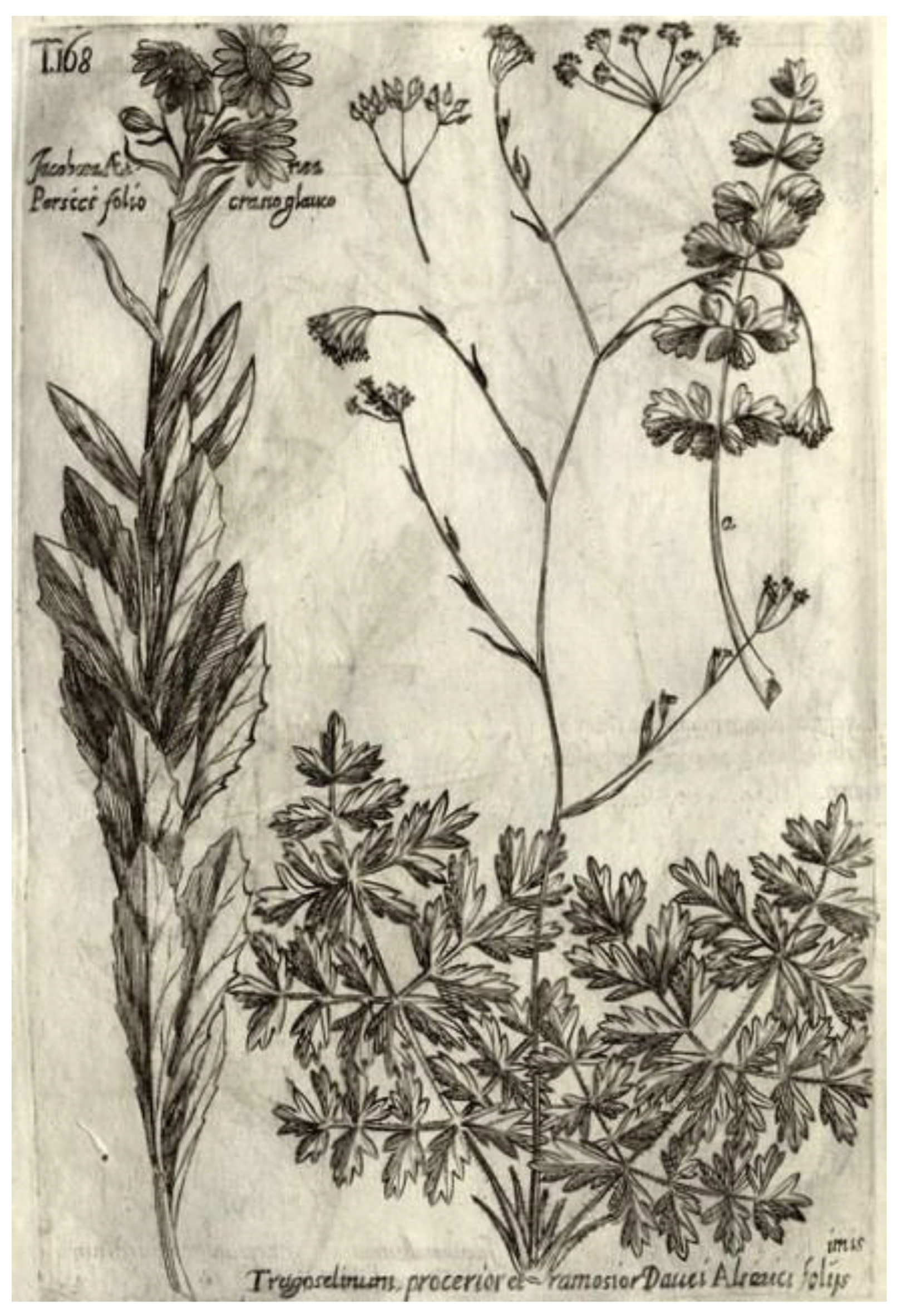The image depicts a delicate, thin cloth or page that could be part of a very old book about plants, resembling a textbook illustration. The material has an off-white, slightly brownish-beige hue suggesting its age. The primary illustration is a meticulous black-and-white or pencil sketch of various flowers and plants, devoid of color. At the top left corner, there is a somewhat unclear text that likely reads "T.108". Surrounding the flowers, there are words in Latin, probably identifying the plant species.

The central floral illustration features three distinct types: On the far left, a tall, slender flower with daisy-like tops extends to the top edge; in the middle, a bushy cluster of leaves supports long, skinny stems adorned with smaller blooms; on the right-hand side, a different plant exhibits a branching structure with leaves and flowers that appear to cascade downwards. Along the bottom edge, additional text can be found, though it's partly illegible. Overall, the drawing looks like a pencil sketch done on fragile, time-worn paper, contributing to its vintage and scholarly aesthetic.